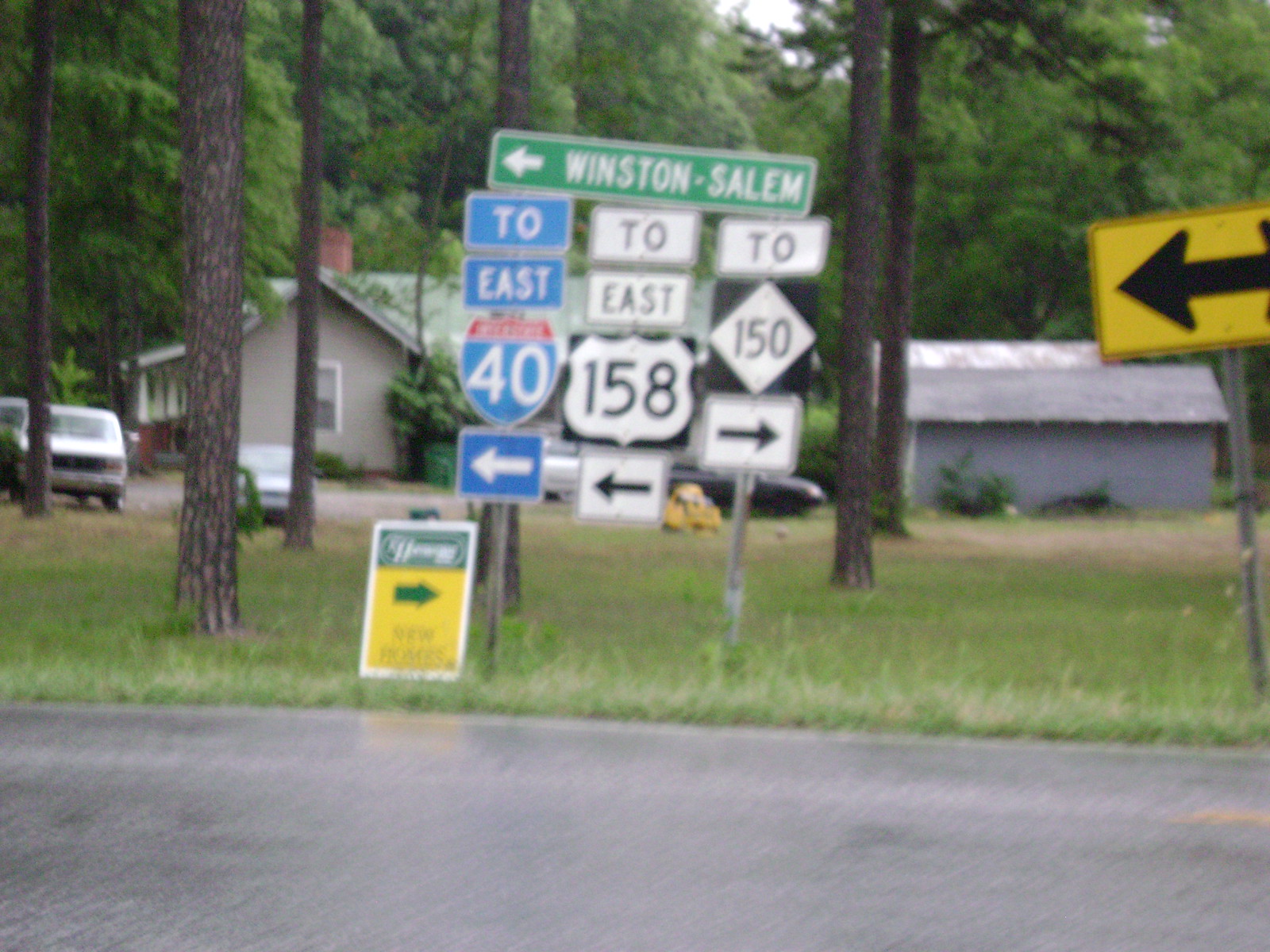The outdoor photograph captures a rural scene centered around a cluster of detailed road signs. The image prominently features a series of directional signs located along a potentially wet, reflective road bordered by dense, tall pine trees and vibrant green grass. In the background on the left side, a gray house with a red chimney is partially visible, nestled among the trees. To the right sits a gray shed, adding to the rural aesthetic. Parked outside the house, two white cars are noticeable.

Dominating the center of the photograph is a bank of road signs. At the top, a green rectangular sign with white text and a left-pointing arrow directs towards Winston-Salem. Below this, three main directional signs indicate different highway routes. The first sign on the left is blue with white text, showing "2 East 40" with a left-pointing arrow. Beside it, a white sign indicates "2 East 158" with a black left arrow. The third sign, also white, reads "2 150" with a black right-pointing arrow. 

Additionally, on the far right edge of the image, there is a yellow rectangular sign with a black bidirectional arrow, suggesting the road reaches a T-junction. A smaller, colorful sign with a green top and yellow bottom appears at the lower part of the sign cluster, likely an advertisement, featuring yellow text and a green right-pointing arrow. The overall composition of the photograph effectively conveys a sense of place and direction within this serene, forested environment.